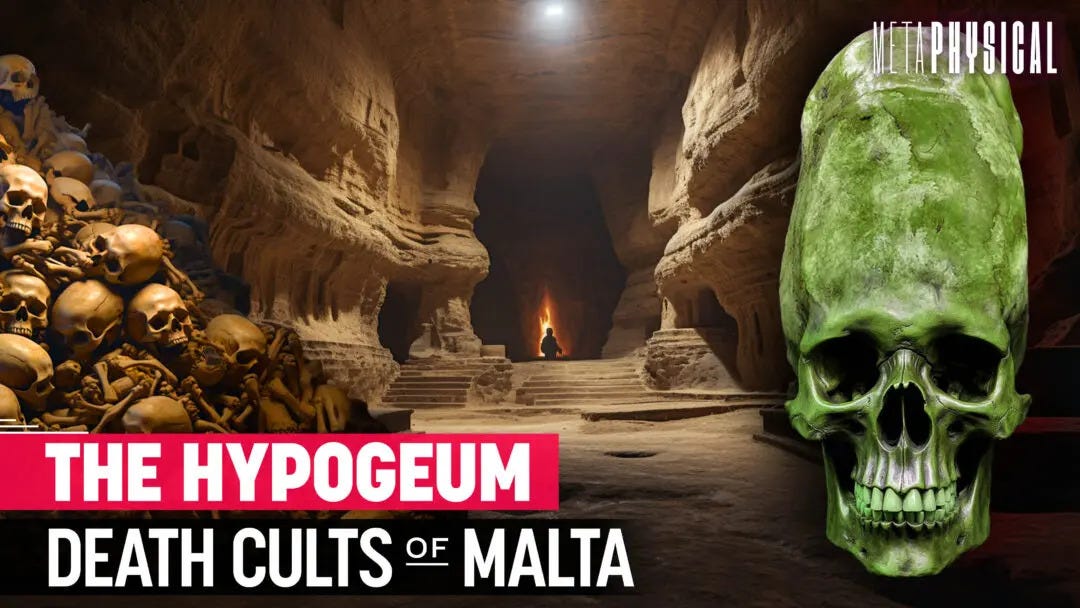The image depicts the interior of an ancient temple or underground cave, with sandstone or dirt stairs leading to a darkened recess illuminated faintly by a distant fire or possible natural light source from above. The temple features carved stone walls and pillars, suggesting an archaeological or haunted ambiance. Dominating the left side of the frame, there's an ominous mound of old skulls and bones, above which a pink banner with large white uppercase letters reads "THE HYPOGEUM." Below this, a black banner states "Death Cults of Malta." On the right side, a strikingly elongated green skeleton stretches towards the top, drawing further intrigue with the word "Metaphysical" inscribed above it. The image, suggestive of a YouTube thumbnail or a promotional shot for a documentary, entices viewers with elements of mystery and the macabre, reminiscent of "Ripley's Believe It or Not."